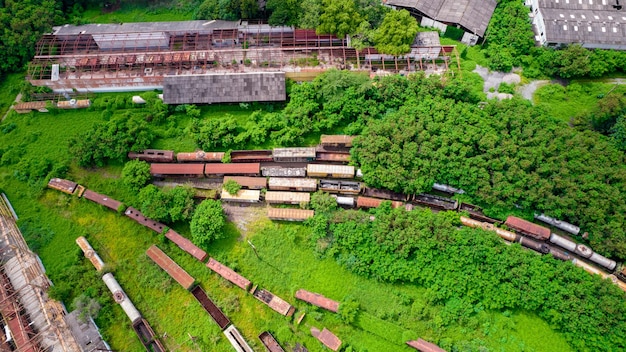This image captures an overhead view of an abandoned train boneyard draped in a lush green forest. In the center of the picture, seven rusted train carriages, in hues of brown, orange, and yellow, extend horizontally from the left to the right, somewhat obscured by encroaching vegetation. The tracks beneath them are barely visible. At the top of the image, the skeletal remains of a long building, with only exposed metal beams where the roof once was, stand as a stark contrast to the greenery surrounding it. On the bottom left, another roofless building frame made of steel is visible. The entire scene conveys a strong sense of abandonment and nature's reclamation, with the once active train yard now overtaken by trees and grass.